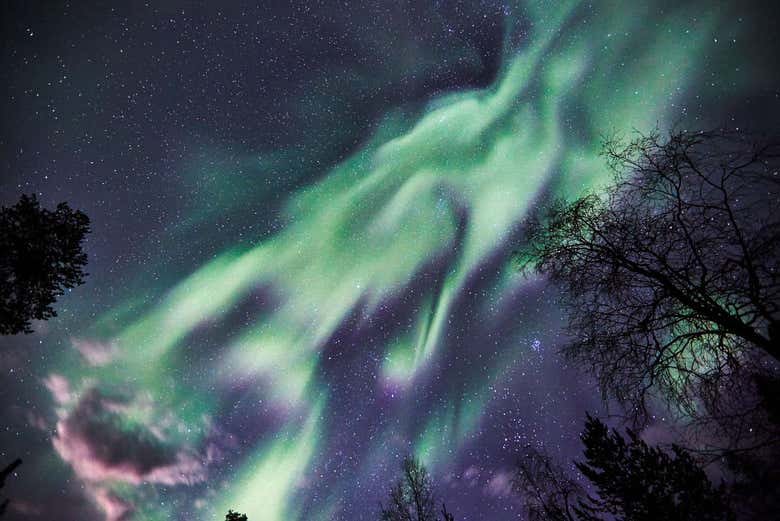This captivating photograph perfectly captures the awe-inspiring beauty of a night sky teeming with stars and the mesmerizing Northern Lights. Viewed from a horizontal landscape perspective, as if lying on the ground or resting your head on a pillow, the image is framed by the silhouettes of various trees along the bottom and sides of the composition. The lower portion features predominantly bare deciduous trees alongside two stately evergreens—the left evergreen extending partway up the frame, while the right one anchors the lower corner.

Dominating the night sky is a breathtaking display of the Northern Lights, intricately woven in soft, swooping lines of green and white that stretch diagonally from the lower left to the upper right. This celestial phenomenon casts a surreal glow across the scenery, and a pinkish tint reflects subtly off fluffy clouds near the lower left corner, adding to the visual symphony. The backdrop is an expansive, dark gray canvas speckled with countless stars, making the sky appear almost infinite. This photograph not only captures the ethereal dance of the aurora but also evokes the profound serenity and wonder of a star-studded night in a tranquil meadow.